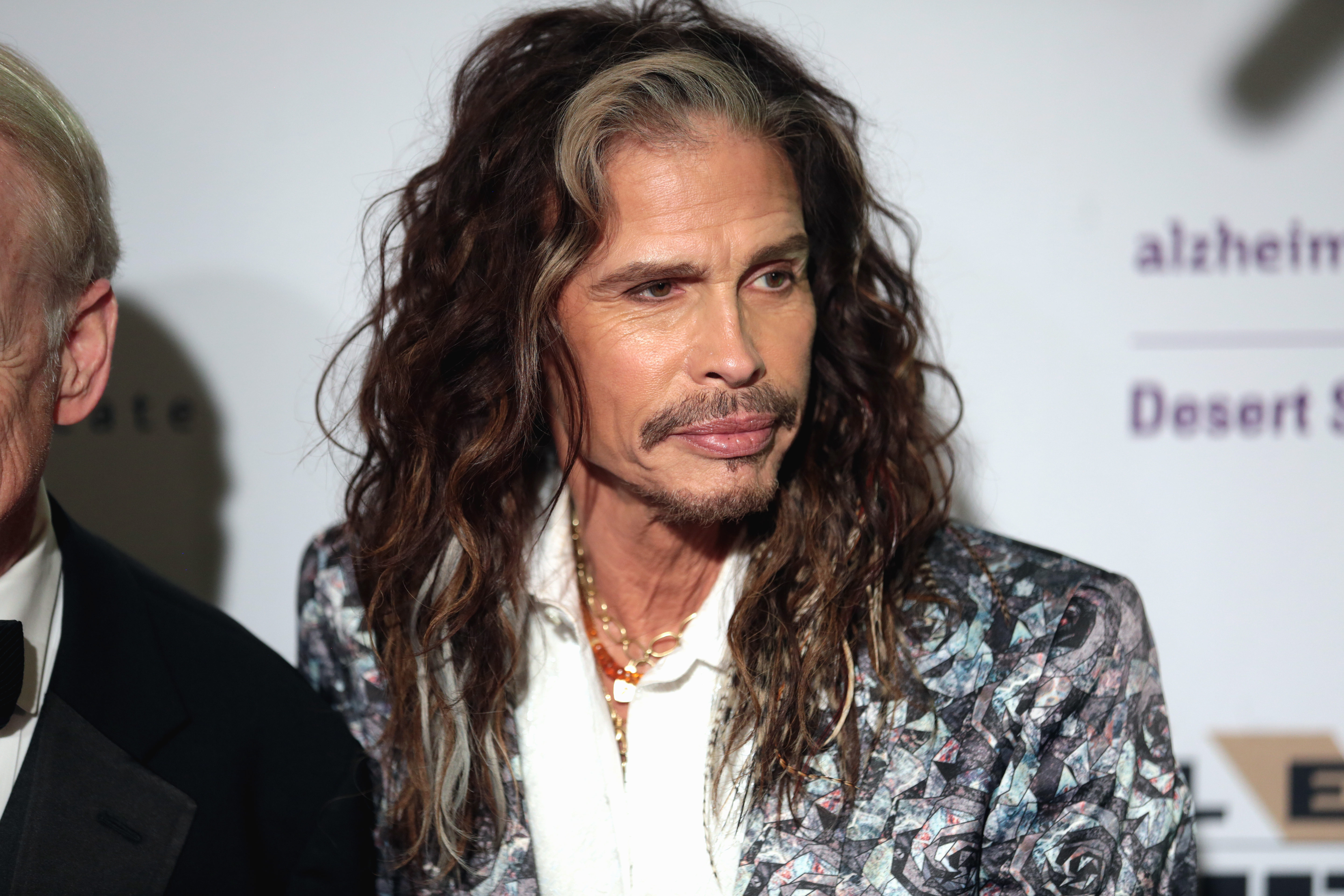In the center of the image stands a renowned rock star, Steven Tyler. His body faces forward and slightly to the left, while his head turns subtly to the right, emphasizing his distinctive profile. His long, brown hair, streaked with whispers of gray, cascades down to his chest. Tyler's facial hair comprises a short mustache and a small beard on his chin. He is clad in a vibrant, multicolored suit jacket adorned with patterns that include hues of blue, pink, white, and black, forming shapes resembling rose buds. Beneath the jacket, he sports a crisp white shirt, partially concealing a gold chain and another indistinct necklace around his neck.

To Tyler's left, another man partially enters the frame. This man, possibly in his 80s, has thin, short, blondish-gray hair and wears a black tuxedo jacket. Visible features include the side of his white shirt collar, a bow tie, part of his left shoulder, and the noticeable wrinkles on his face. The background reveals a plain white wall with the partially visible text "ALZHEI...," presumably referring to Alzheimer's, followed by "DESERT" and a line of text that extends beyond the image's edge.